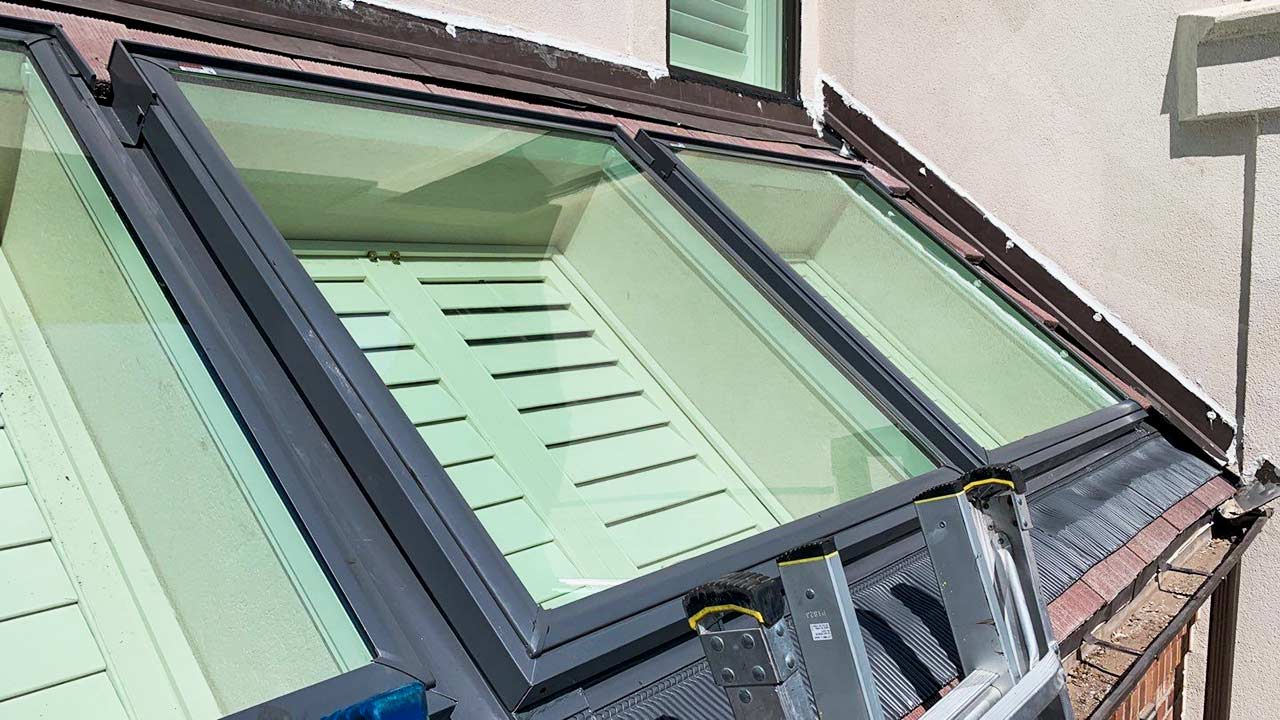In this image, three skylights are prominently featured, each framed in grey and fitted with clear glass. These skylights, which are used for natural lighting and temperature control, have internal wooden panels in a lime green hue that are currently closed. The skylights are evenly spaced along the upper part of the structure, which has a slight pinkish tint at the very top. Surrounding the skylights is grey flashing, with black flashing situated just below them. To the right side of the image, a white stucco wall is visible. Adjacent to the wall, leaning against the black eavestrough, is a silver-grey ladder. The ladder has small black rubber tips at the top edges for grip and protection. Just above the stucco wall to the left, green panels can be seen behind another glass surface, contributing to the image's layered architectural details.